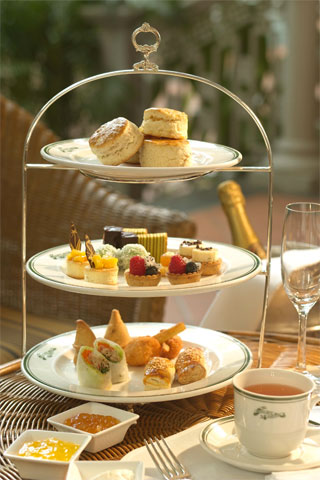This image captures an elegant tea time setup, highlighted by a prominent three-tiered silver metal plate holder adorned with a key design at the top. The top tier features four round biscuits, while the middle and bottom tiers display an assortment of small pastries, cookies, and possibly some bite-sized sandwiches wrapped in pita, all arranged on white plates with delicate, possibly floral designs. A white porcelain teacup with a textured design, filled with what appears to be yellowish tea, is situated in the lower right corner of the table. Beside it sits a silver fork and a pair of small square dishes containing various jams or marmalades, as well as a third dish that looks like it might contain mayonnaise. On the table's left side, there's a crystal champagne flute, either empty or filled with water, with the top of a champagne bottle peeking out from a bucket behind the three-tiered stand. The entire arrangement rests on a wicker table, and a hint of wicker furniture is visible in the muted background, suggesting an outdoor setting. The refined and beautiful presentation creates a sophisticated ambiance perfect for a leisurely tea or dessert time.